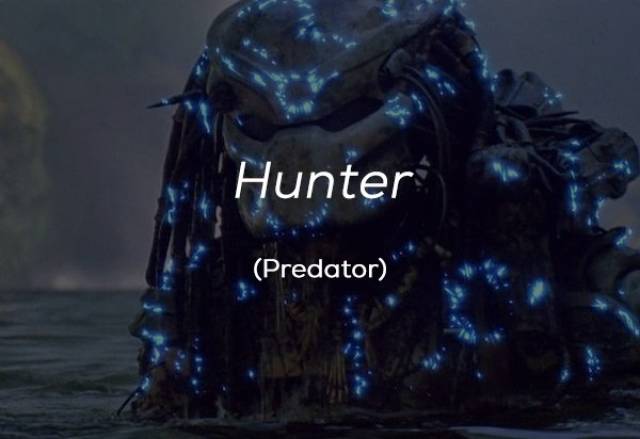The image is a screenshot from the movie "Alien vs. Predator." Dominating the center to the right side of the picture is a black alien—distinctively a predator—emerging from murky, dark water that lacks visible waves. This water extends across the lower portion of the image, creating an ominous setting enhanced by the dark, grayish-black sky in the background. The predator, with light-blue neon lights accentuating various parts of its grey, shiny, possibly wet skin, has a triangular head that dips towards a pointed nose, and sports long, hair-like dreadlocks hanging from its skull-like helmet, down to its shoulders. The creature appears to be slightly glowing, adding to its eerie presence. Overlaying the central part of the image, in bold white letters, the text reads "Hunter," followed by "Predator" just beneath it. The predator gazes downwards to the right, adding to the intense and foreboding atmosphere of the scene.